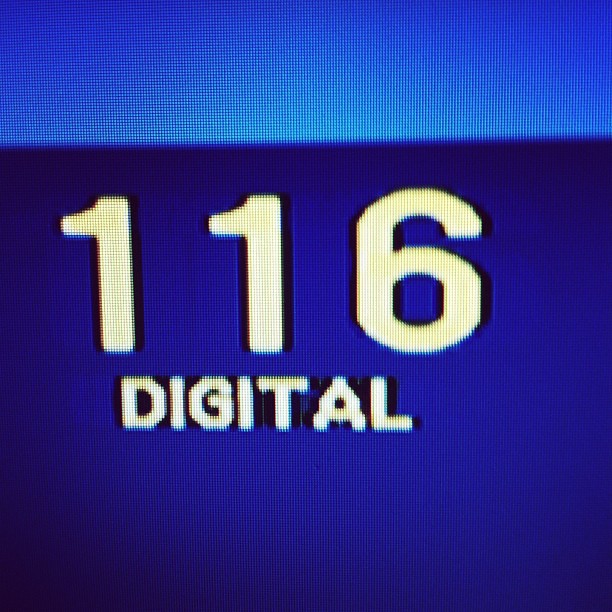This is an up-close photograph of a digital screen. The top quarter of the image is a light blue color, clearly separated by a darker blue line from the rest of the image, which is a deep, dark blue. In the center, the number "116" is prominently displayed in large white text, with both "1"s having pointed tips. Below the number, the word "DIGITAL" is written in all capital letters, also in white. Both the number and the word "DIGITAL" are highlighted by black borders. When viewed closely, the image reveals fine black horizontal and vertical lines indicative of individual pixels, emphasizing that the photo is a depiction of an electronic display, possibly an older computer screen or a digital measuring device.